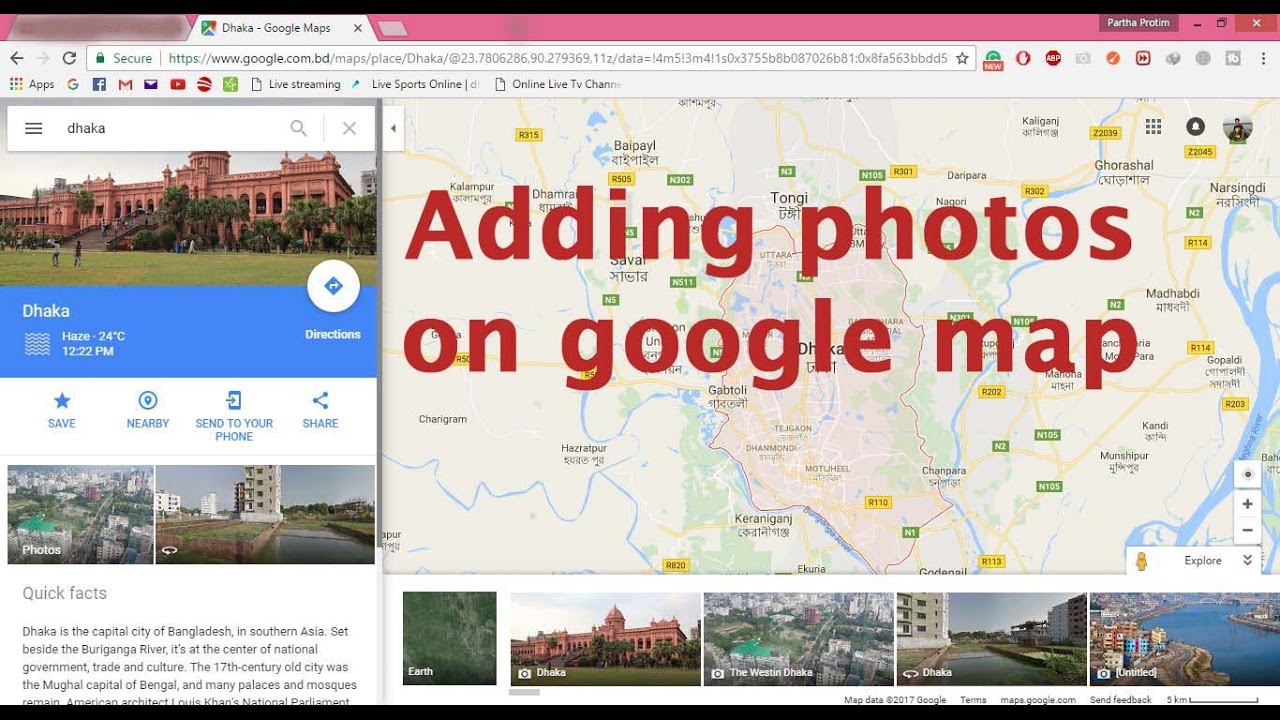This is a detailed screenshot of a Google Maps interface showing the location of Dhaka. The screenshot prominently displays a picturesque monument, a significant and beautiful building, possibly a historic site. The display indicates current weather conditions in Dhaka, noting that it's hazy with a temperature of 24 degrees Celsius at 12:22 PM. 

The interface features several functionalities such as saving the location, searching for nearby points of interest, sending the location to a phone, or sharing it. Additionally, there are photos of the area and a brief informational section under "Quick Facts". This section describes Dhaka as the capital city of Bangladesh, located beside the Buriganga River. It highlights Dhaka's historical significance, pointing out that the city was the Mughal capital of Bengal in the 17th century and retains many palaces and mosques from that era. Notably mentioned is the National Parliament designed by American architect Louis Kahn, although the text cuts off at this point.

The screenshot also shows instructions for adding photos on Google Maps, suggesting it might be part of a tutorial or guide on how to navigate and interact with the map, including uploading images. The overall presentation offers a comprehensive view of the location along with the various features available for interacting with the map.